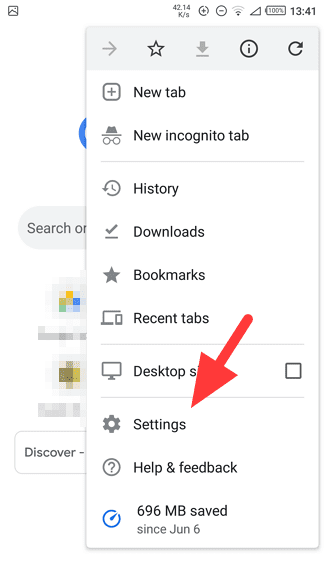This screenshot, taken on a cell phone, captures an open options window located in the top right-hand corner of the screen. The window, which has a white background and black text, lists the following options: New Tab, New Incognito Tab, History, Downloads, Bookmarks, Recent Tabs, Desktop Site, Settings, Help and Feedback, and Data Savings. Specifically, the image indicates that 696 MB of data have been saved since June 6. A red arrow prominently points to the Settings option within this menu.

In the background, the slightly pixelated and blurry page appears to be open to the Google search engine homepage, where a portion of the search bar is visible, displaying the word "Search." Additionally, in the very top right-hand corner of the screen, the time is shown as 13:41, with the battery indicator displaying 100% charge.